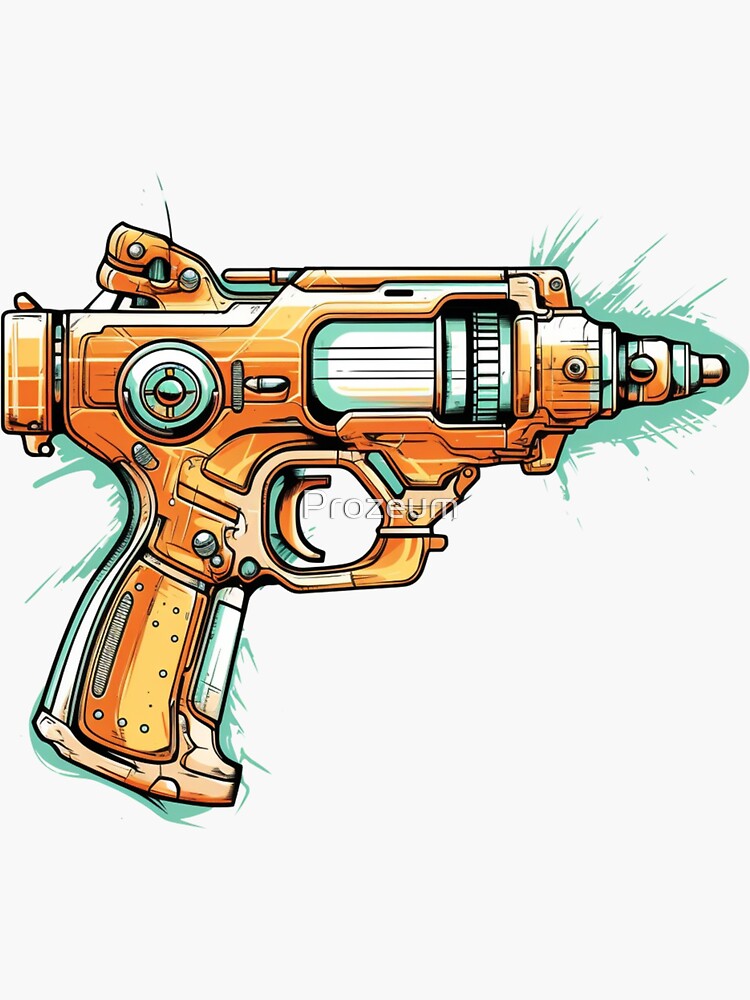This digital graphic depicts a detailed illustration of a futuristic orange ray gun, prominently featuring a blend of both playful and advanced design elements. The gun, which lacks a traditional barrel, is equipped with a knob-like tip suggesting it emits a laser rather than bullets. The body, predominantly orange and boldly outlined in black, includes intricate internal mechanics visible through a cutaway section. These mechanics likely involve a spinning wheel mechanism to generate laser energy. Accents of light green and aqua hues decorate the handle and muzzle, adding a dynamic painted effect. The image is set against a rectangular, light gray background with the gun centered and pointed to the right. The image also features a semi-translucent watermark reading "PROZOUM" or "Prosium" in white and gray, adding a distinctive touch to the artwork.